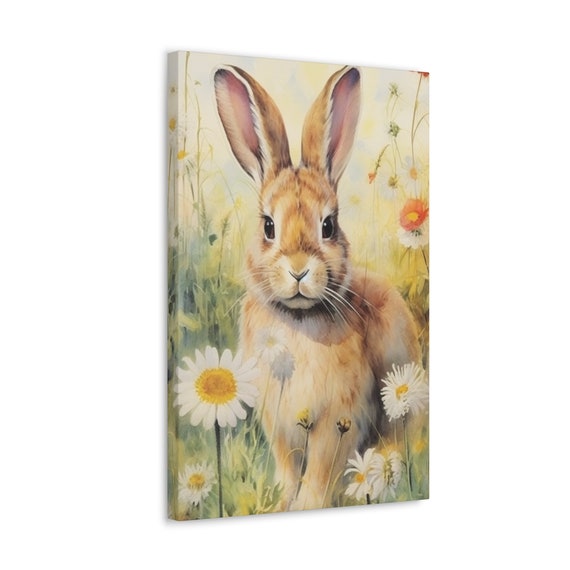This detailed canvas painting portrays an endearing light brown and tan bunny rabbit, distinguished by its large, upright ears revealing delicate pink interiors and complemented by expressive dark brown eyes. The artist masterfully depicted the fine texture of the bunny's fur, with individual hairs artistically sketched to create a realistic, dynamic visual. The bunny, with its white whiskers and small tan nose, is shown in a vertical stance, looking intently at the viewer, creating a sense of direct engagement. Set amidst a vibrant field of wildflowers, the scene features daisies with yellow centers and white petals, alongside other colorful blooms, including pinkish-red flowers. The lush green grasses and multi-hued floral tips add depth and richness to the background. A soft, glowing yellow sky in the backdrop suggests sunlight gently bathing the scene, enhancing the tranquil and picturesque ambiance of the artwork.